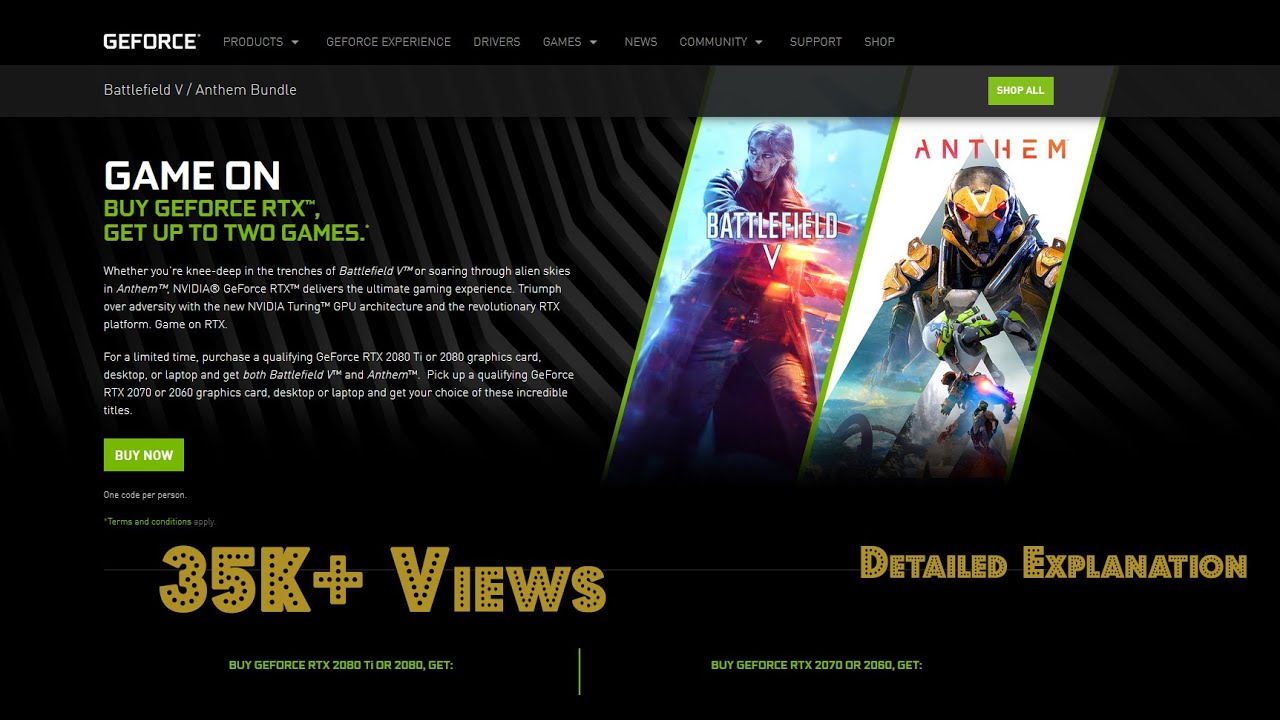This image is a detailed snapshot of the GeForce website interface. At the top of the page, users are presented with navigation options, including "Products," "Before Experience," "Drivers," "Games," "News," "Community," "Support," and "Shop." Prominently displayed in the center is the Battlefield vs. Anthem bundle.

The central focus is on a promotional offer where users can get up to two games, showcased under the banner "Game On by GeForce RTX." To the right, two promotional images are displayed diagonally from right to left, representing the games Battlefield V and Anthem. Each image features characters: Battlefield V showcases soldiers, whereas Anthem features mechanized combat suits.

Below the images, there's a descriptive section detailing the offer. A "Buy Now" button is prominently located for easy access. Furthermore, the page highlights that the promotional content has been viewed over 35,000 times. Additional options are available to the right, including a "Detailed Explanation" link.

At the bottom of the promotional section, users are provided with choices to either "Buy GeForce RTX 2080 DET" or click on "Buy Before," separated by a vertical line for clarity.